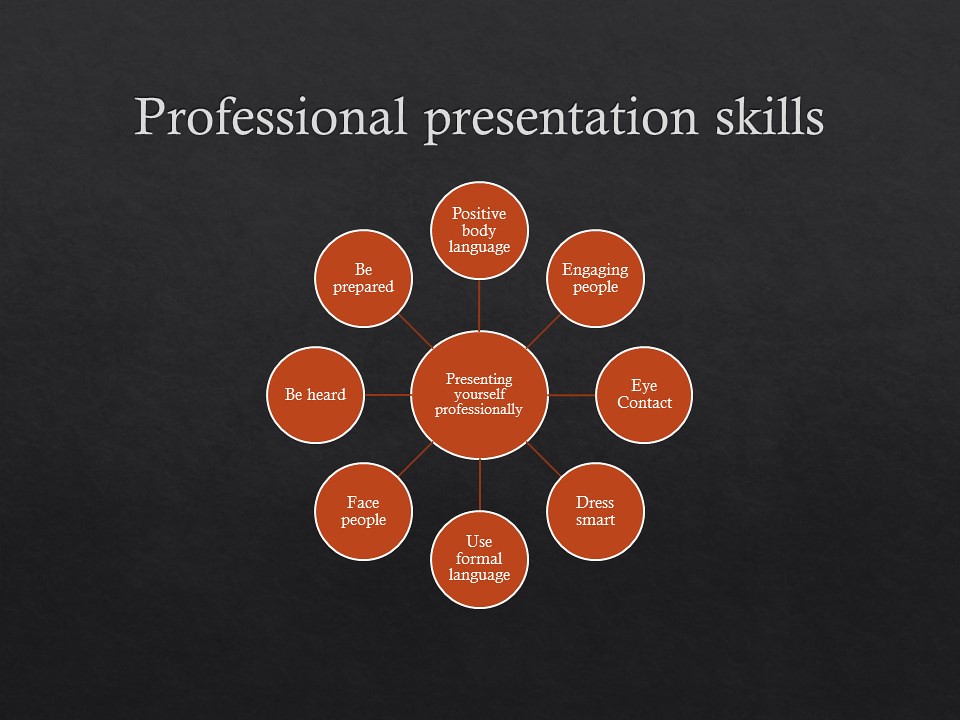The image features a dark black background with white text at the top that reads "Professional Presentation Skills." Centrally, there is an orange chart with multiple circles radiating out from a main circle. Each circle is connected by red lines and outlined with a white border. At the center, the largest circle states "Presenting Yourself Professionally." Surrounding it, in clockwise order, the smaller circles are labeled with presentation skills: "Positive Body Language," "Engaging People," "Eye Contact," "Dressing Smart," "Use Formal Language," "Face People," "Be Heard," and "Be Prepared." This detailed illustration serves as a comprehensive guide to mastering professional presentation skills.